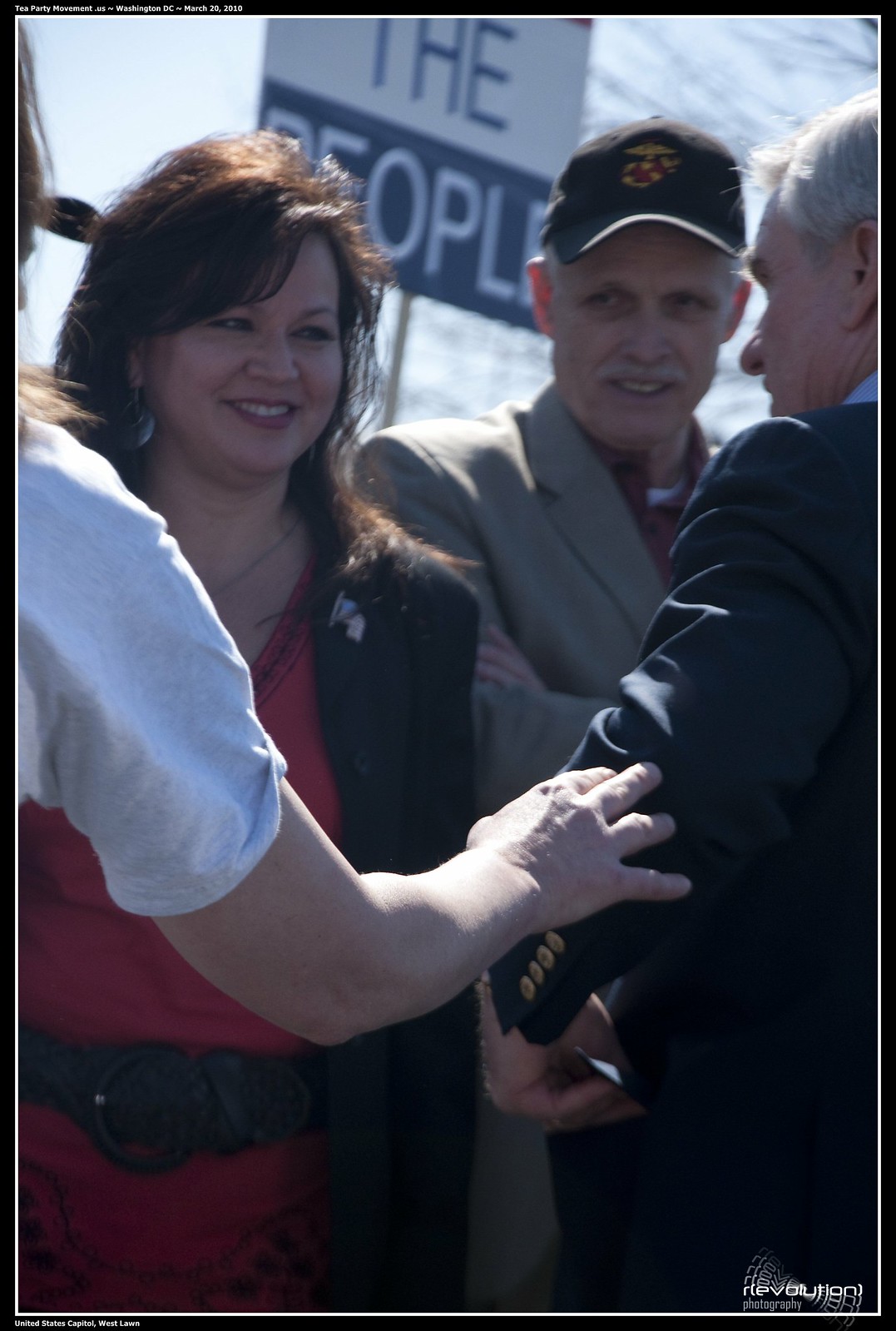The photograph captures a lively outdoor scene where a group of people appears to be engaging with a female politician, likely campaigning or promoting her election. The central figure is a Latino woman in her 40s, wearing a red dress with a black jacket adorned with an American flag pin. She has dark hair that falls to her shoulders and engages animatedly with the people around her.

Next to her on the right stands an older man in a brown jacket and blue baseball cap, with a white mustache that adds a distinguished touch to his appearance. On the far right edge of the picture, another older man can be partially seen, dressed in a dark suit with white hair peeking from the side.

In the background, a blue and white sign is visible, with the words "the people" discernible, suggesting a political or public gathering. The scene is lit by natural daylight, reflecting off the crowd's heads, and framed by a gray sky and bare tree branches, indicating a chilly fall or spring day.